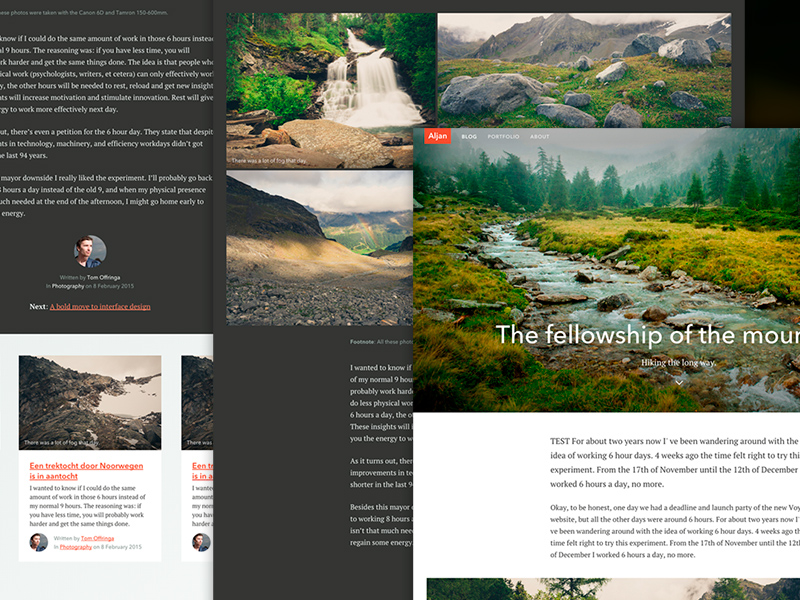A serene landscape featuring a cascading waterfall flowing into a crystal-clear creek is surrounded by lush green grass. In the background, majestic mountains rise with imposing gray rock formations, while patches of snow rest on black rocks to the left. The scene is peppered with vibrant yellow and green grass, adding a touch of color to the verdant setting. Further downstream, another creek winds its way through tan dirt and more scattered black rocks both above and below. In the midst of this picturesque scenery, a backhoe loader stands, possibly used for some recent construction or maintenance work. Amidst the natural elements, a profile picture of a man with short dark hair is also displayed with the name "Al Jan." The mention of "the fellowship of the Mau" suggests a unique group or theme linked to the setting.